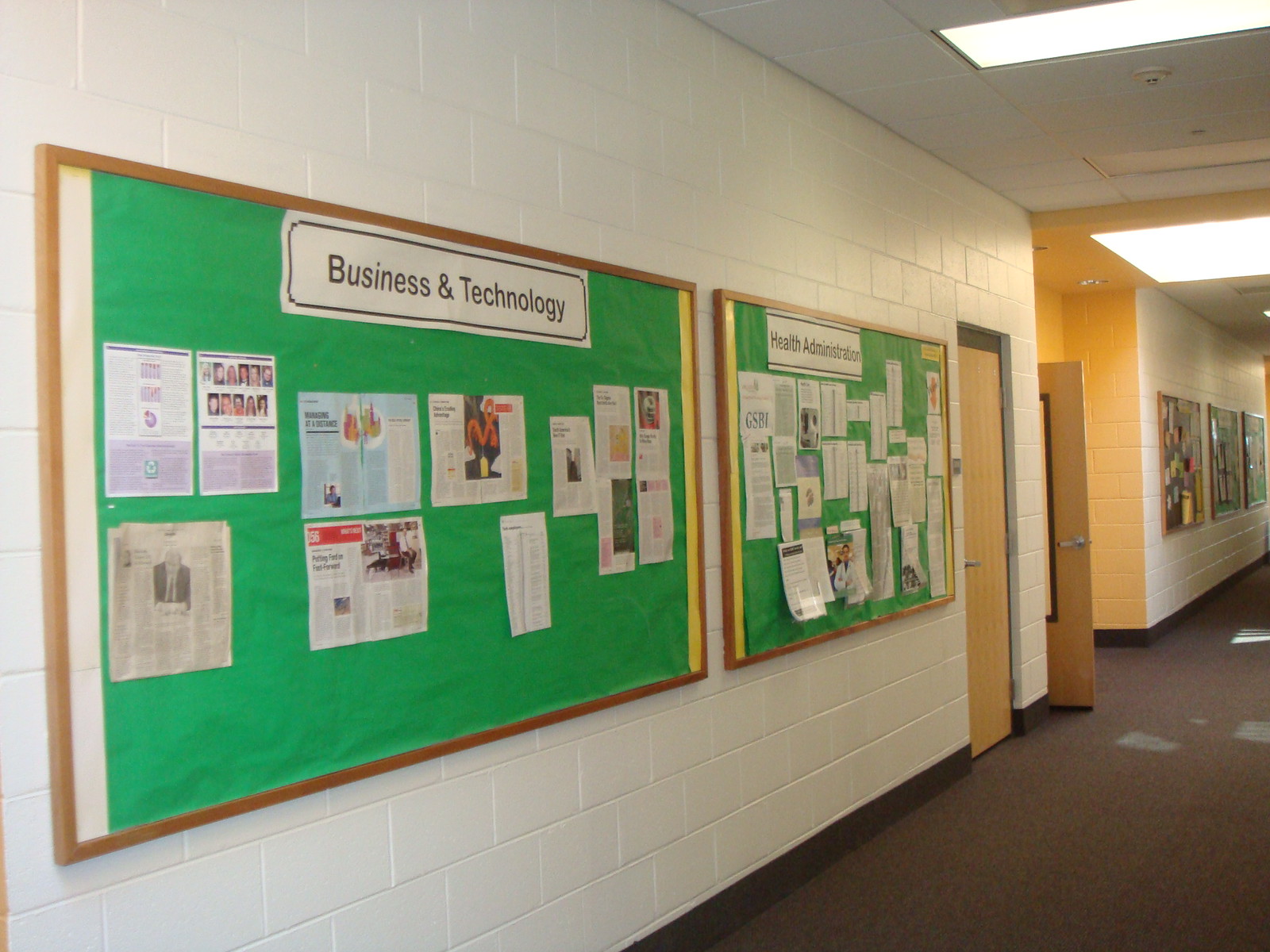The image depicts a school hallway at an angle, featuring a mix of brown and gray carpeting and white painted cinder block walls with black trim at the bottom. The ceiling is fitted with tile panels and square light fixtures. Dominating the left side of the wall is a light wooden door, next to which there is an open door in an alcove. Prominently displayed along the hallway are large cork bulletin boards with green backgrounds. The nearest board is labeled "Business and Technology" and is covered with various newspaper clippings, magazine pages, and journal cuttings related to those fields. Further down the hall, there's another board titled "Health Administration," which holds roughly twice as many articles. At the far end of the hallway, three more bulletin boards are visible, though the details of their contents cannot be discerned.